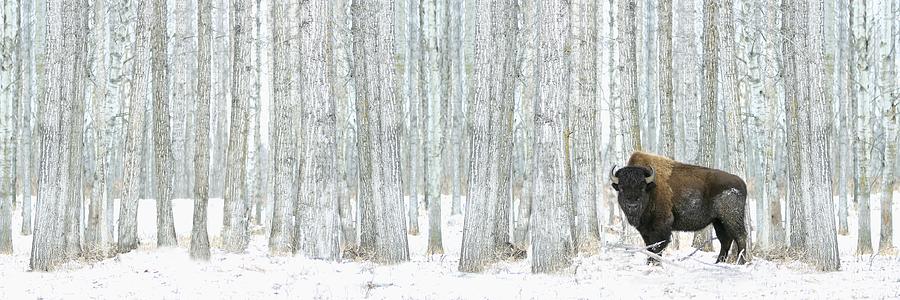The image is a panoramic winter scene featuring a dense forest and a solitary American bison. The snowy forest floor is punctuated by around fifty trees of varying diameters, from slender young trunks to thicker, mature ones, arrayed in rows that stretch across the long, narrow photograph. The scene is imbued with hues of black, gray, light blue, and light green, lending it a surreal, almost painterly quality. On the right third of the image stands the bison, its large frame covered in shades of dark and light brown. Snow clings to its flanks and belly, and its horns are visible. The bison gazes pensively toward the camera, as if posing for the shot, its presence the only sign of life in this tranquil, snow-draped setting. The sky beyond the grove of trees is a faint, light blue, adding to the serene atmosphere of the wintery tableau.